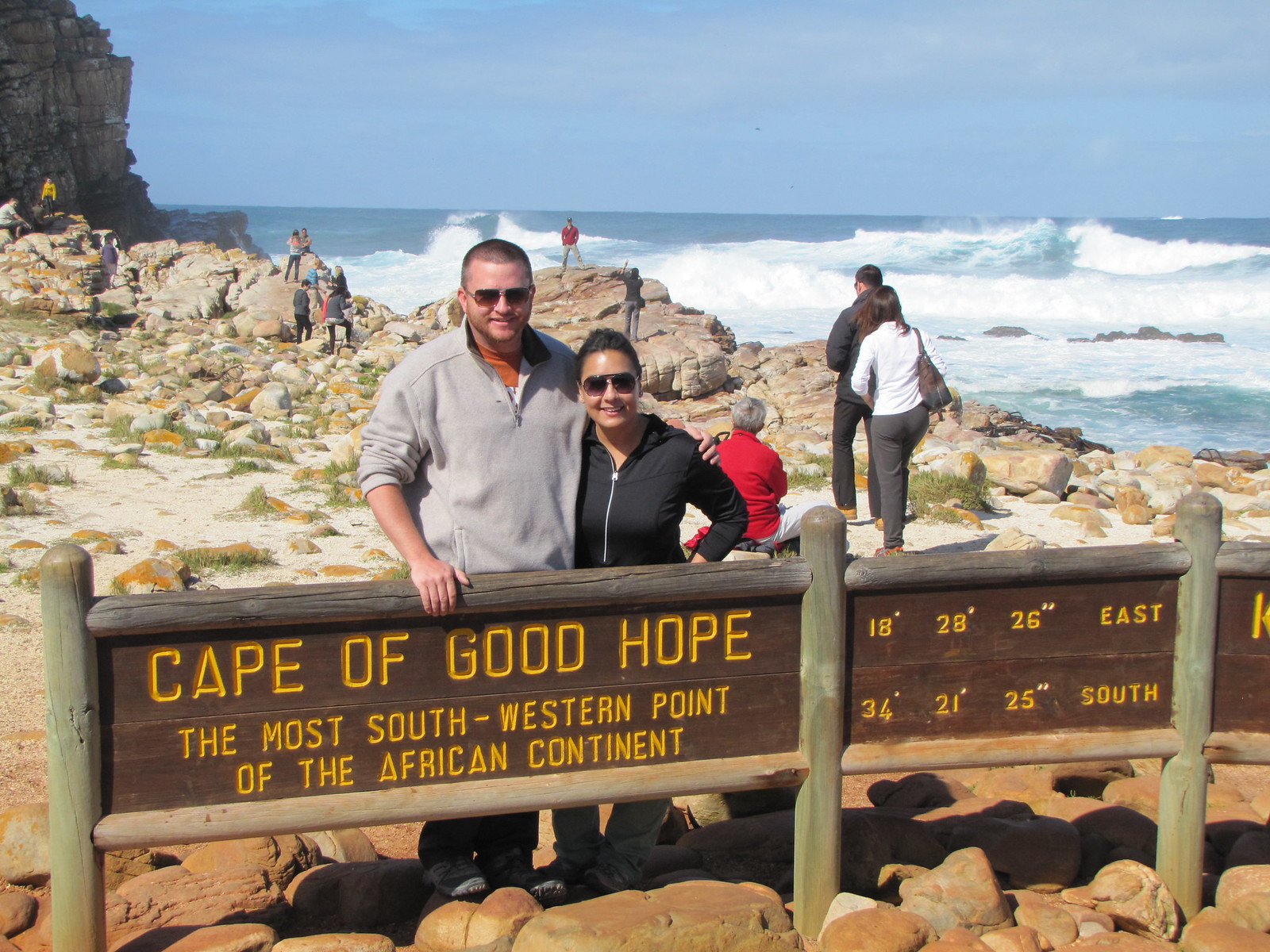The photograph captures the scenic Cape of Good Hope, renowned as the most south-western point of the African continent. The image is bustling with activity; a couple stands front and center, posing for the camera. The man, clad in a gray sweater over an orange shirt and sporting sunglasses, stands beside a woman in a black hoodie with a zipper and black sunglasses. They both appear to be tourists, enjoying the picturesque setting. Behind them, several people are exploring the rocky terrain that stretches to the ocean, where white waves and bubbles froth upon the water's edge. Dominating the scene is a sturdy wooden sign with thick logs supporting it. The sign, with a dark brown background and bright yellow text, proclaims: "Cape of Good Hope, the most south-western point of the African continent." Coordinates are displayed on the right side of the sign, reading "18, 28, 26 east" and "34, 21, 25 south." The environment features large rocks to the left, and the expansive blue sky beautifully frames the idyllic coastal landscape.